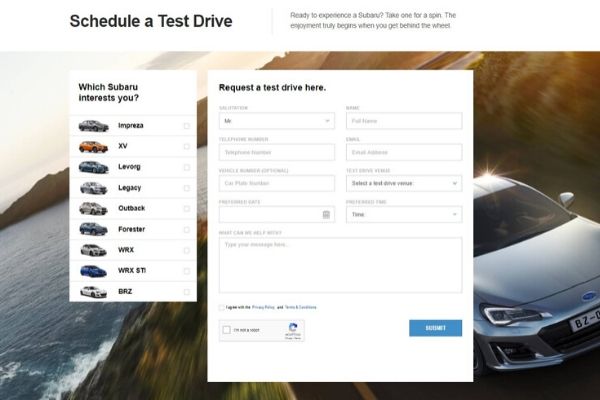The image depicts a computer screen displaying a Subaru website dedicated to scheduling test drives. At the very top, written in bold black font, are the words "Schedule a Test Drive." Below this header, there's a column with the title "Which Subaru Interests You?" suggesting this page is intended for selecting different Subaru models for a test drive, whether sponsored by the dealer or the company itself.

On the right side of the screen, fine print reads, "Ready to experience a Subaru? Take one for a spin." At the center of the image, a prominent box labeled "Request a Test Drive Here" contains fields for entering your name and relevant information, along with a CAPTCHA check at the bottom left to verify user authenticity.

The background of the website features a scenic image: to the left, part of a serene lake is visible, set against a mountainous backdrop to the right. The foreground displays the front half of a gray Subaru, with a glint of sunlight reflecting off its top surface. The license plate partially reads "BZ."

Additionally, the left side of the screen lists various Subaru models, including the Ingress and XV, with a total of nine or ten different models available for selection for a test drive.